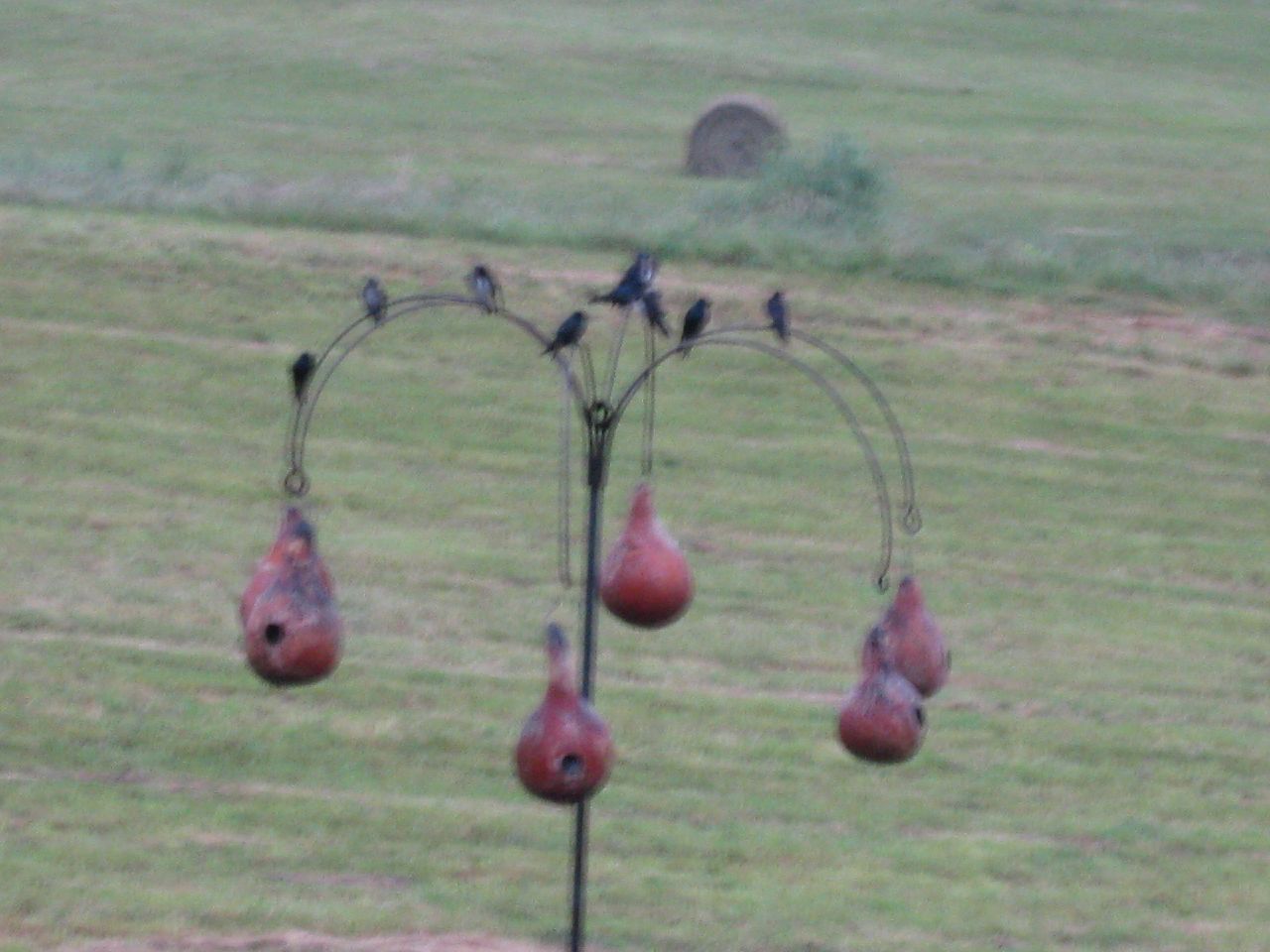This landscape-oriented photograph captures a vibrant scene set in verdant green fields, with lush grass and a ball of brown hay visible in the background. Dominating the center of the image is a distinct artificial tree-like structure with a sturdy black rod anchored firmly into the ground. Atop this main rod are five evenly spaced, flexible, and curved branches, each adorned with hooks suspending gourd-shaped birdhouses. These birdhouses have a rustic burgundy hue and feature a distinct hole at the front, resembling potential nesting sites for birds. Perched atop the structure are about eight black birds, possibly preparing to enter these inviting avian homes. The thoughtful placement and detailed craft of the structure, combined with the pastoral landscape, create a harmonious sanctuary for the birds amidst the natural beauty of the farmland.